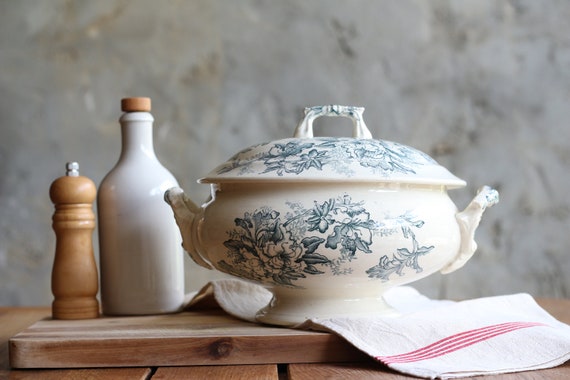In this photograph, positioned on a wooden surface, we see a detailed arrangement centered around a striking crockery item. This item, which appears to be a substantial teapot, is predominantly white with intricate black designs in the shape of leaves and flowers, giving it an elegant chinoiserie appearance. The teapot is equipped with two side handles and a top handle on its round lid, indicating it is made of porcelain. Placed underneath this teapot is a white cloth adorned with classic red stripes.

To the left of the teapot stands a white bottle, likely intended for olive oil, contributing to the overall domestic scene with its simple design. Adjacent to this bottle is a brown object that resembles a chess piece, probably functioning as a salt and pepper shaker. The background reveals a grey concrete wall, adding a neutral contrast to the scene. This composition reflects a blend of functional kitchen items and decorative elements, suggesting a well-used and cherished collection of items on the wooden table.